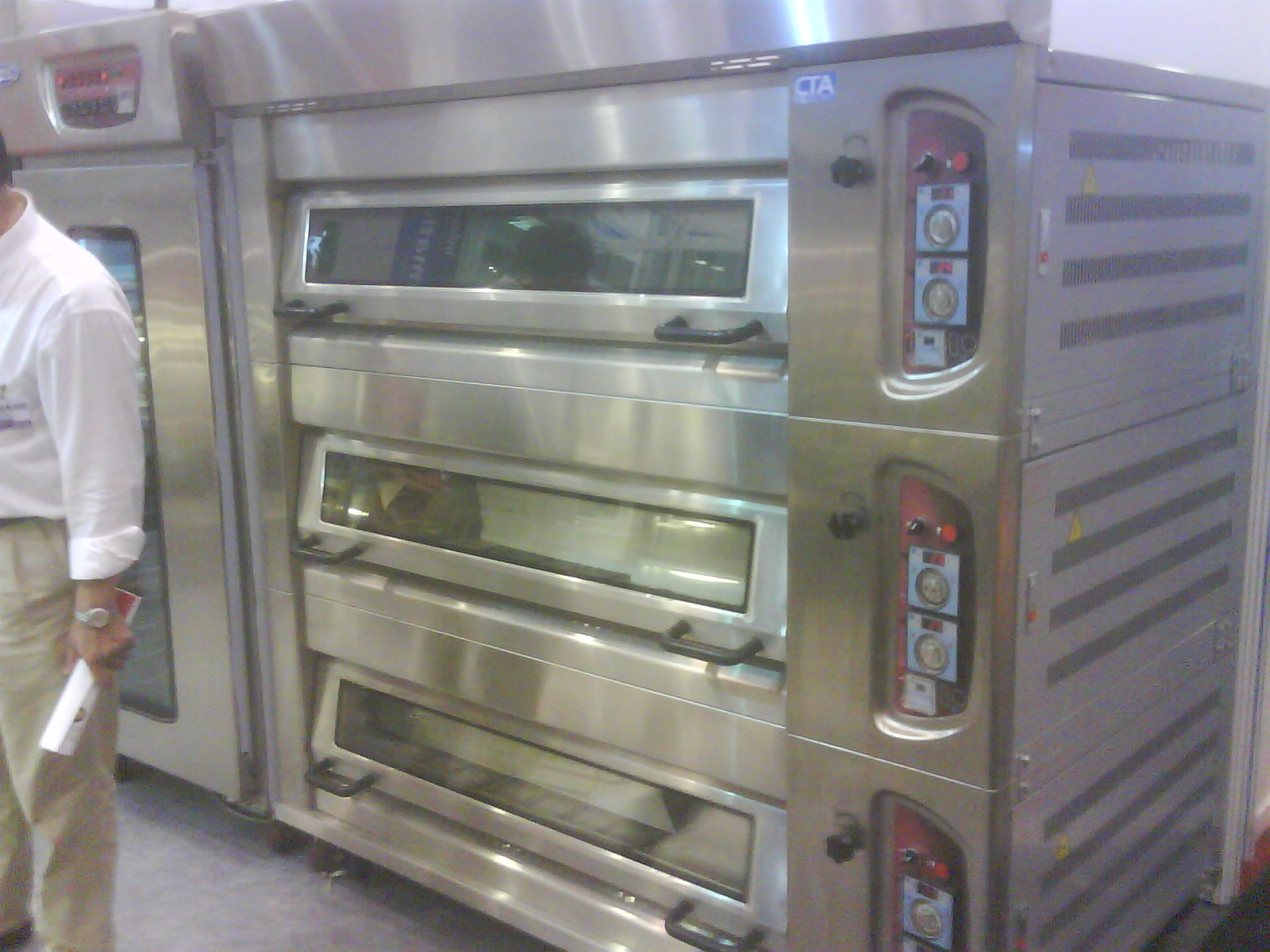The image portrays a large, industrial-grade machine, likely an oven or scientific device, that dominates the entire frame from top to bottom. This metallic apparatus, possibly stainless steel, features three identical sections stacked vertically. Each section includes a long rectangular glass window with two black handles on either side. The control panels on the right of each section have a greenish tint and are equipped with various buttons, including red and black knobs, and a couple of blue squares with red text. The logo "CTA" is prominently displayed in the top left corner of each panel, outlined in blue. The floor beneath the machine is gray, reflecting the utilitarian setting.

On the left side of the image, a man is partially visible, with only half of his body in the frame. He has dark hair and is dressed in a white, long-sleeve shirt with rolled-up cuffs and khaki pants. His left arm hangs by his side, holding a rolled-up piece of paper or booklet that is white with some red markings. The man's watch is also visible, adding to the detailed portrayal of his attire. The industrial and somewhat clinical ambiance is strongly suggested by the shiny, chrome-like finish on the machine and the visible functionality of the control panels.